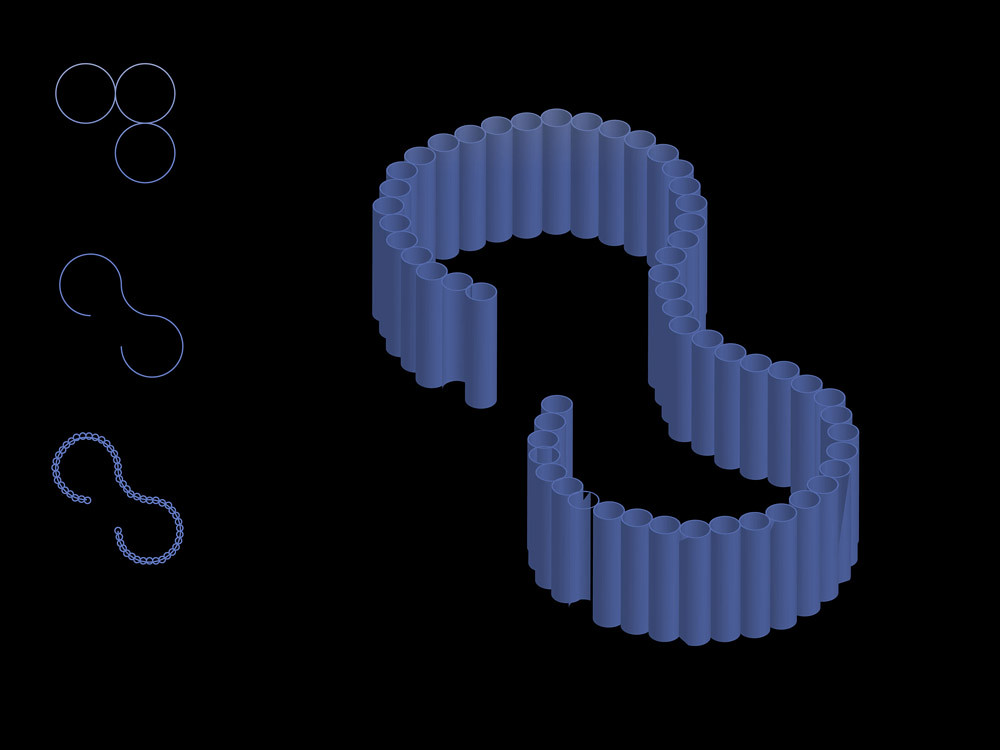This image features a series of interconnected geometric shapes set against a deep black background. In the upper left corner, three circles of identical size are arranged with two side by side and a third directly beneath the rightmost circle. Below this trio, a white, curved line resembling a sideways number three is displayed vertically, evoking the image of a squiggle. This shape appears again directly beneath the squiggle, this time resembling a chain link fence in texture and form. Central to the composition is a three-dimensional version of this squiggle-like figure, comprising an intricate structure of small white tubes arranged vertically to form the shape.